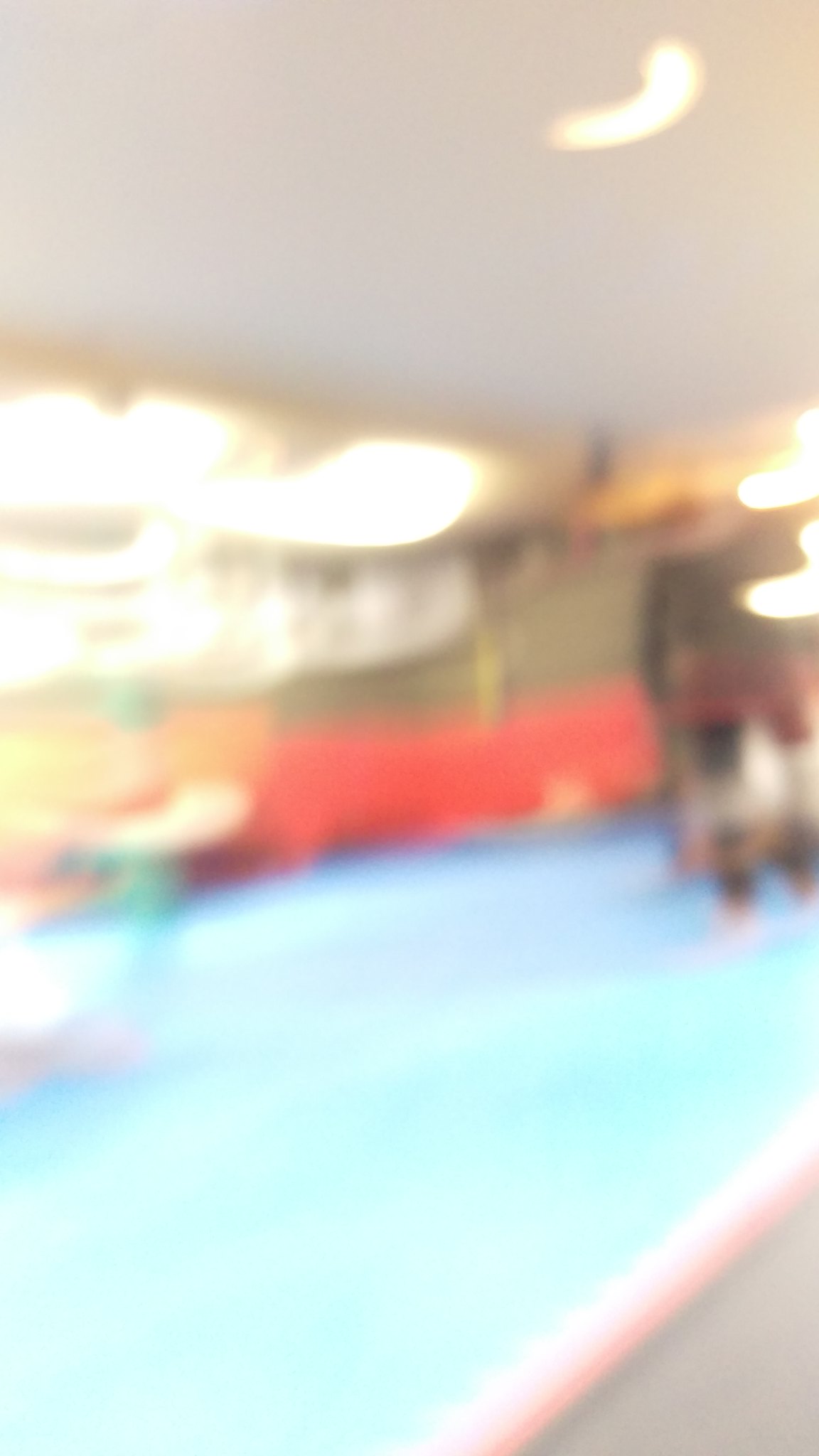This vertically-aligned, extremely blurry photograph appears to have been taken indoors, possibly in a waiting room. At the top of the image, there is a ceiling with can lights and other fixtures that cast light on the scene. The background features a red area, likely benches or seats, indicating it could be a public space. The floor is notably blue, which might initially resemble water but is confirmed to be a solid surface. On the right side stands a figure, possibly in a darker outfit, and may be wearing red shorts. This individual is likely an African American adult, and their presence suggests the scene is not underwater. Additionally, there is a vertical element on the left side of the image that could be a pole or column. The ceiling and walls are cream beige, contributing to the overall interior atmosphere.